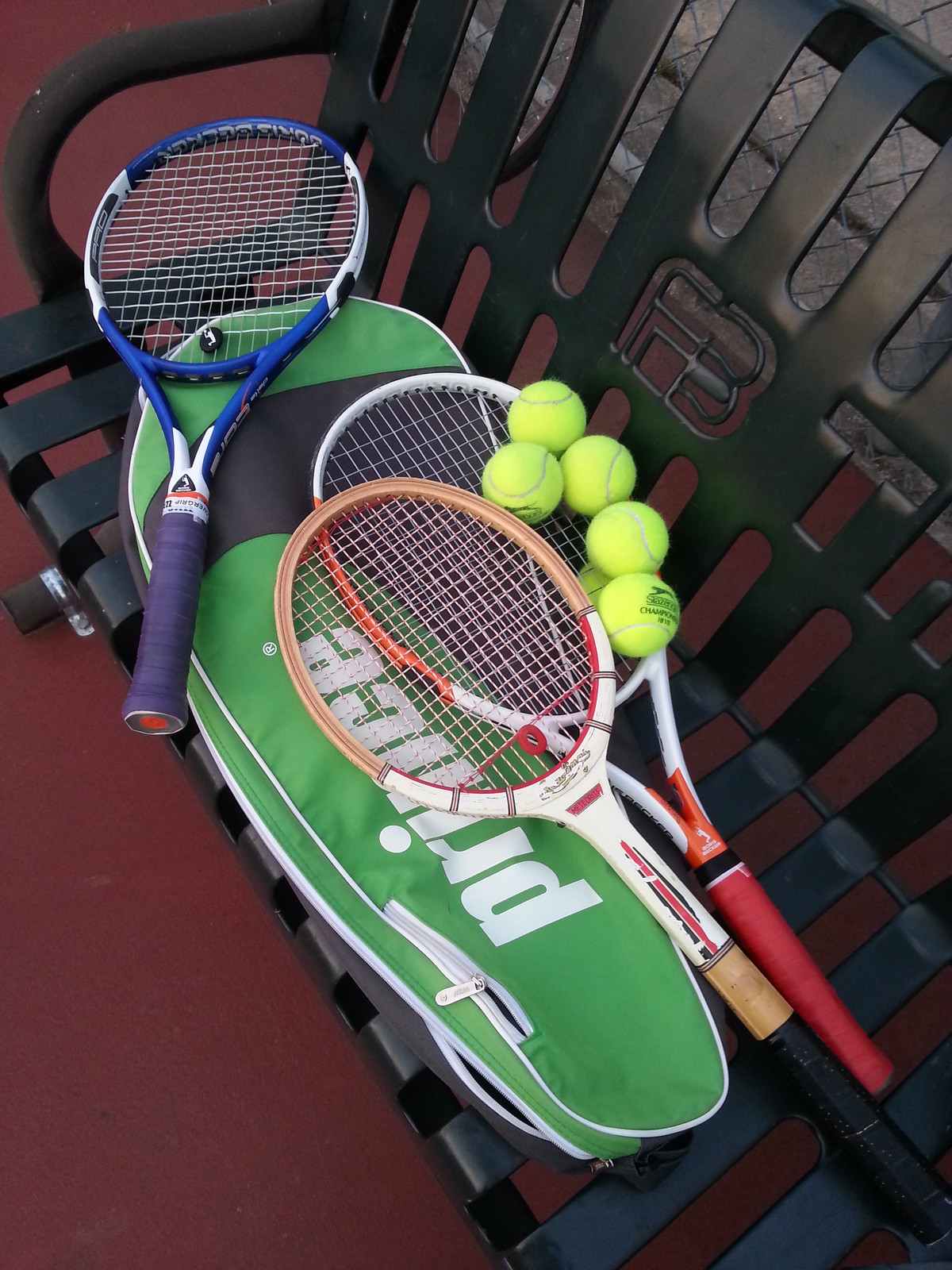This color photograph depicts three tennis rackets and a green racket bag with the brand name "Prince" in white letters. The rackets and bag are laid out on a black park bench situated on a tennis court, identifiable by the court's distinctive surface. The tennis rackets display a range of colors and designs: the top racket features a blue handle and frame, the bottom racket that holds five tennis balls has a red handle with a white frame, and the leftmost racket has a wooden frame and a long black handle. Additionally, one description mentions a reddish floor and a room, but the dominant details point to an outdoor tennis court setting for this scene.